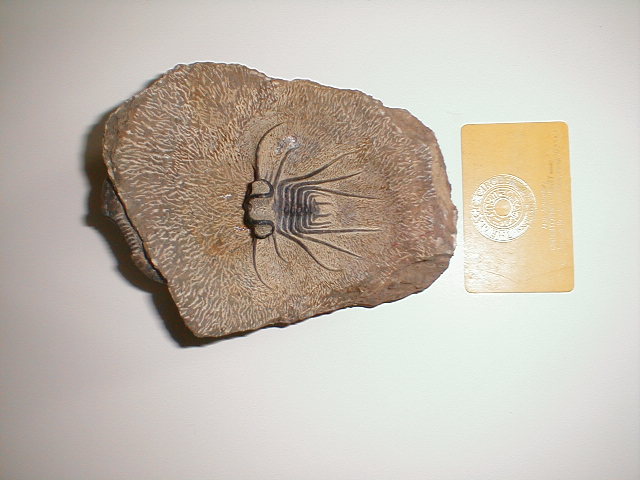The image shows a detailed fossil specimen, resembling a brown, somewhat flat and wavy-edged piece of petrified wood or rock, prominently featuring a well-preserved insect at its center. The insect, possibly a large beetle or mosquito, is almost the same size as the petrified piece and appears to be fossilized within it, showcasing intricate details such as segmented body parts, antennae, numerous legs, and a pair of wings. To the right of the fossil is a yellow card, about the size of a credit card, possibly indicating the scale of the specimen, and the entire scene is set against a stark white background.